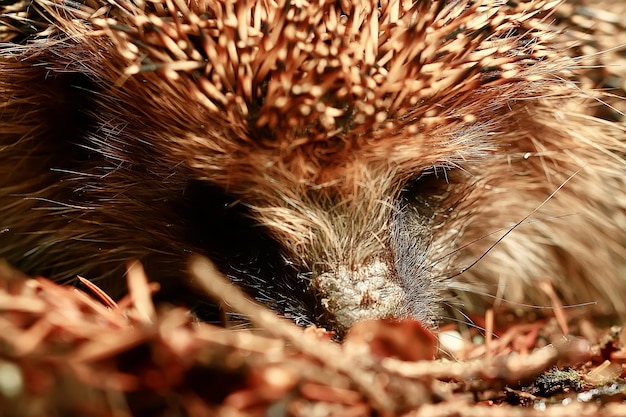This is a detailed close-up of a porcupine's face, capturing its distinctive features with a focus on the nose, eyes, and whiskers. The porcupine's nose is blunted and covered in thick hair, while long grayish-whitish whiskers extend from the nose-cheek area. Its eyes, which are a recessed dark brown, give the appearance of being somewhat hidden against the similarly colored ground. The top of its head shows a mixture of pointy quills in black, brown, and beige shades, blending seamlessly with the gray and beige tones of its fur. The porcupine appears to be laying amidst twigs, leaf debris, and foliage, making it almost camouflaged against the similarly colored background. Only the face and top of the head are visible, with long hair on the sides giving a prickly yet soft appearance. The image evokes a sense of curiosity as the porcupine seems to be either eating, smelling, or simply observing its surroundings.